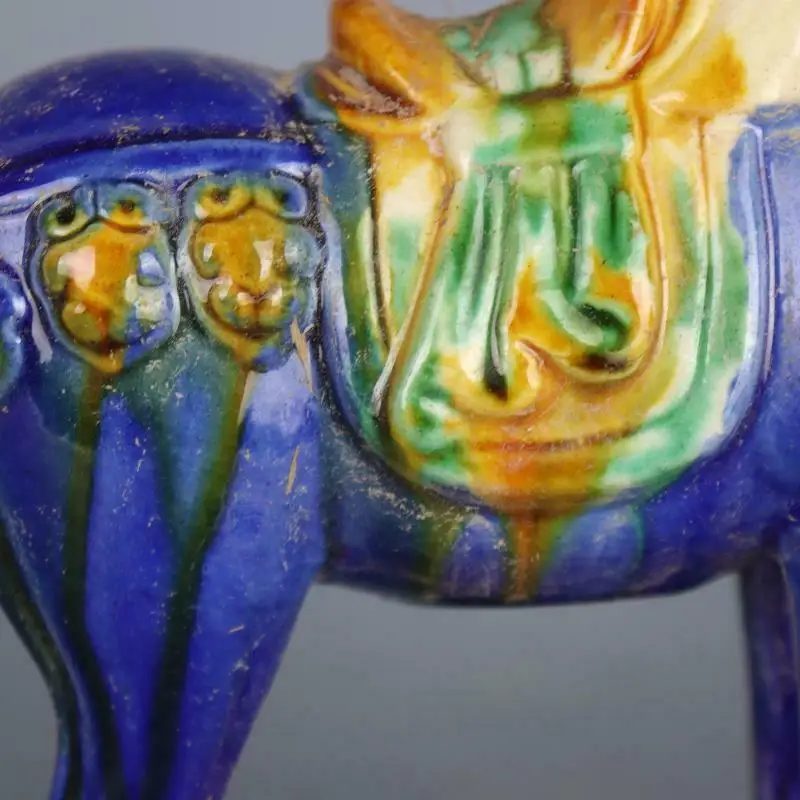The image shows a detailed ceramic statue of a horse and rider, primarily focusing on the midsection and hind legs of the horse. The horse is a striking blue color with green stripes running down its back legs. The rider appears to be a polo player, as indicated by the visible hockey stick-like object and the rider's legs hanging down. The statue does not reveal the horse's head, but a significant decorative element is present near the horse's back hip.

The saddle is richly colored: the parts where the rider's feet rest are green, transitioning to an orange seat, and yellow hues towards the front. These colors blend together, giving the saddle a melted, dynamic look. The rider’s feet are surrounded by green, and there's an artistic representation of the rider’s head integrated into the saddle design. This intricate ceramic piece captures the elegance and dynamic movement of a horse in mid-gallop, reflecting both artistry and attention to detail.